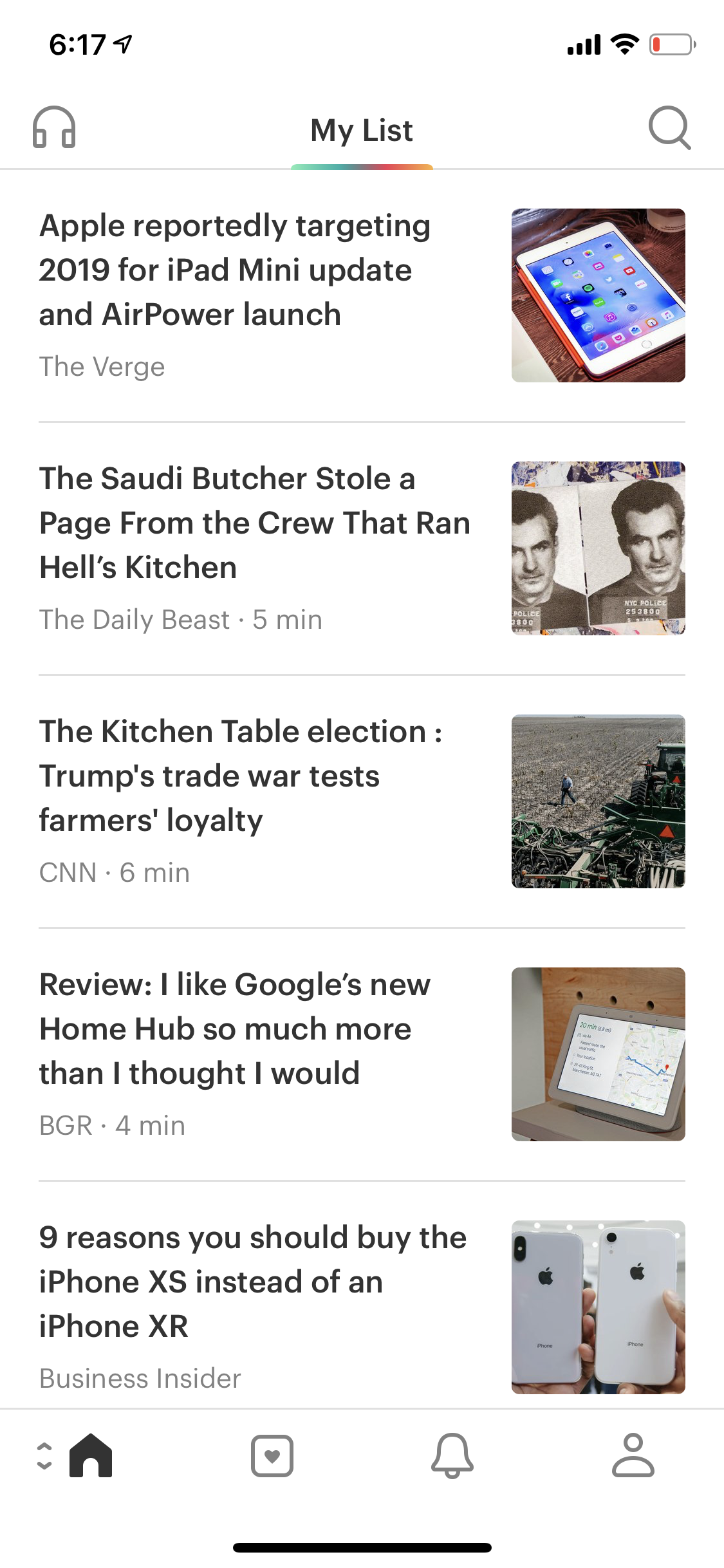A detailed screenshot displayed on a user's smartphone shows a news application interface. At the top of the screen, the time is displayed as 6:17. The battery icon, located on both the top left and right corners, is in red, indicating it is almost depleted. The device has a strong connection, with all five signal bars fully lit. Below these icons, on the left, there is a headphone icon, and on the right, a magnifying glass icon representing the search function.

In the center of the screen, the highlighted and underlined title "My List" indicates that this section is active. The vertical list below it features various news articles from different sources, each accompanied by a corresponding image to its right.

The first article from The Verge is titled "Apple reportedly targeting 2019 for iPad mini update and AirPower launch," with an image of an iPad beside it. The second article from The Daily Beast reads "The Saudi butcher stole a page from the crew that ran Hell's Kitchen," complemented by a photo showing the Saudi butcher in a double image format. The third article, titled "The kitchen table election: Trump's trade war tests farmer's loyalty," depicts a large open field with a farmer and heavy machinery to his right. Next, a review article titled "I like Google's new Home Hub so much more than I thought I would" features an image of a laptop displaying Google's Home Hub. The final article from Business Insider is titled "Nine reasons you should buy the iPhone XS instead of an iPhone XR," though an image is not explicitly mentioned in the provided text.